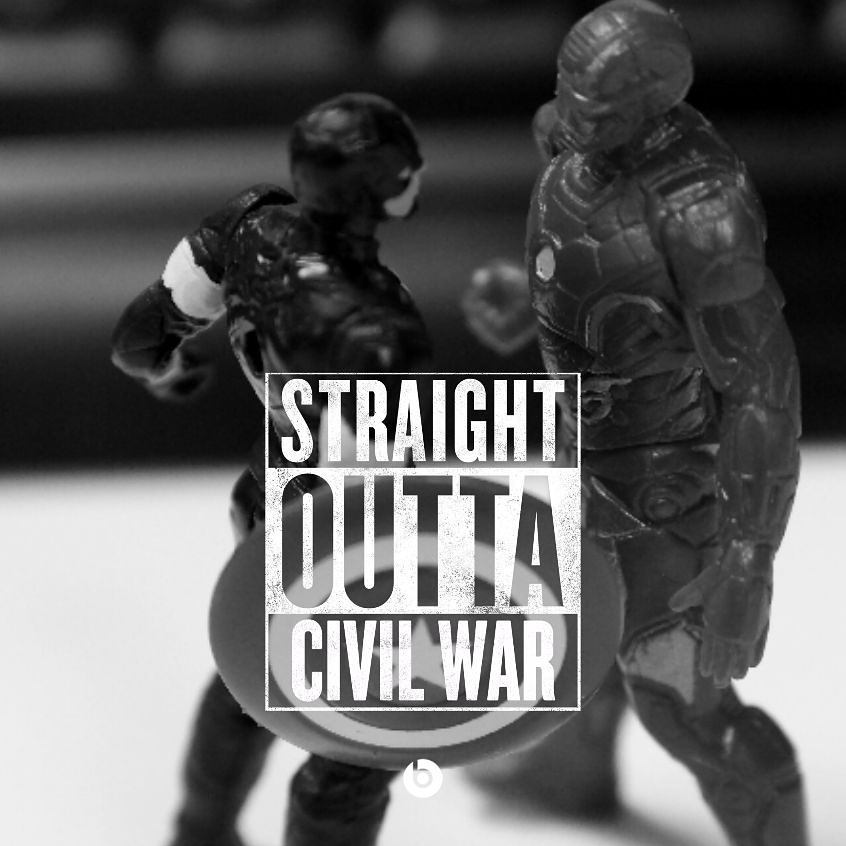This detailed black and white photograph captures two action figures, positioned to mirror an iconic scene from Marvel's movie "Captain America: Civil War." The left figure, unmistakable as Captain America due to his shield, faces slightly to the right, his pose indicating readiness for confrontation. Opposite him on the right is Iron Man, identified by the distinctive shape of his armor, posed in a stance echoing an impending clash. Both figures stand on a light-colored, slightly blurred surface that fades out at their ankle level, adding to the dramatic tension of the scene.

Superimposed on the image is a white-outlined text box, primarily overlaying Captain America's right arm and his shield. The box features layered text that reads "straight" at the top in white letters, followed by "OUTTA" in red with a semi-transparent background revealing the figures behind it, and finishes with "Civil War" in white at the bottom. This text, resembling a digital watermark, underscores the central theme of the photo, paying homage to the film's epic battle between the two legendary superheroes. The background at the top of the image is purposefully blurred, keeping the focus squarely on the heroic showdown.